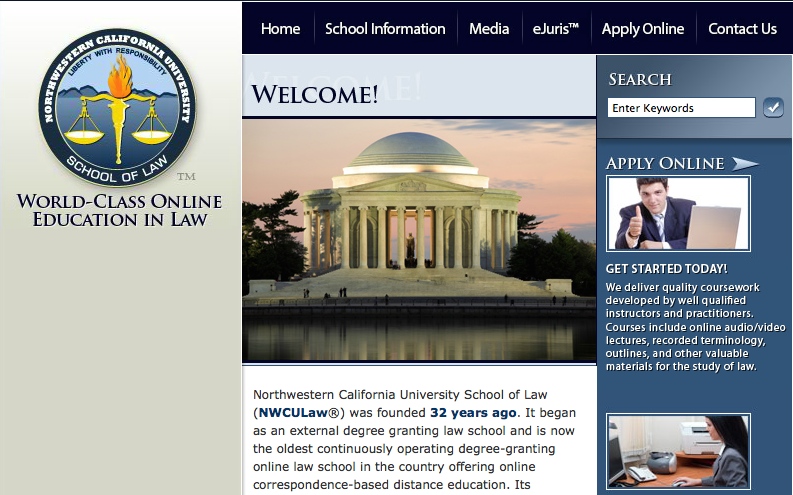This is a landscape-oriented photo, slightly longer than it is tall, depicting a webpage related to a law school affiliated with a university. The photo features a black border across the top but no other surrounding borders. 

On the left side of the photo, there is a vertical column showcasing the logo of Northwestern California University, which consists of a set of scales with a flame, accompanied by the motto "Liberty with Responsibility." Below the logo, it states "School of Law," with "World Class Online Education and Law" inscribed in blue font beneath it.

To the right, at the top of the image, there's a black background housing clickable white links. The navigational links, from left to right, are: "Home," "School Information," "Media," "eJuris," "Apply Online," and "Contact Us."

Beneath these links, there is a light blue banner that reads "Welcome!" with an exclamation point and a white shadow effect. To the right of this banner is a search box labeled "Enter Keywords."

The main section of the photo features an image of a stately, pillar-fronted capitol building. To the right of this building, there's another light blue box with the header "Apply Online." This box includes a picture of a man in a suit giving a thumbs up with his right hand while seated at a laptop. The accompanying text says "Get Started Today" in white, followed by a description.

At the very bottom of the page, it reads "Northwestern California University of Law," followed by a brief description of the institution's history.